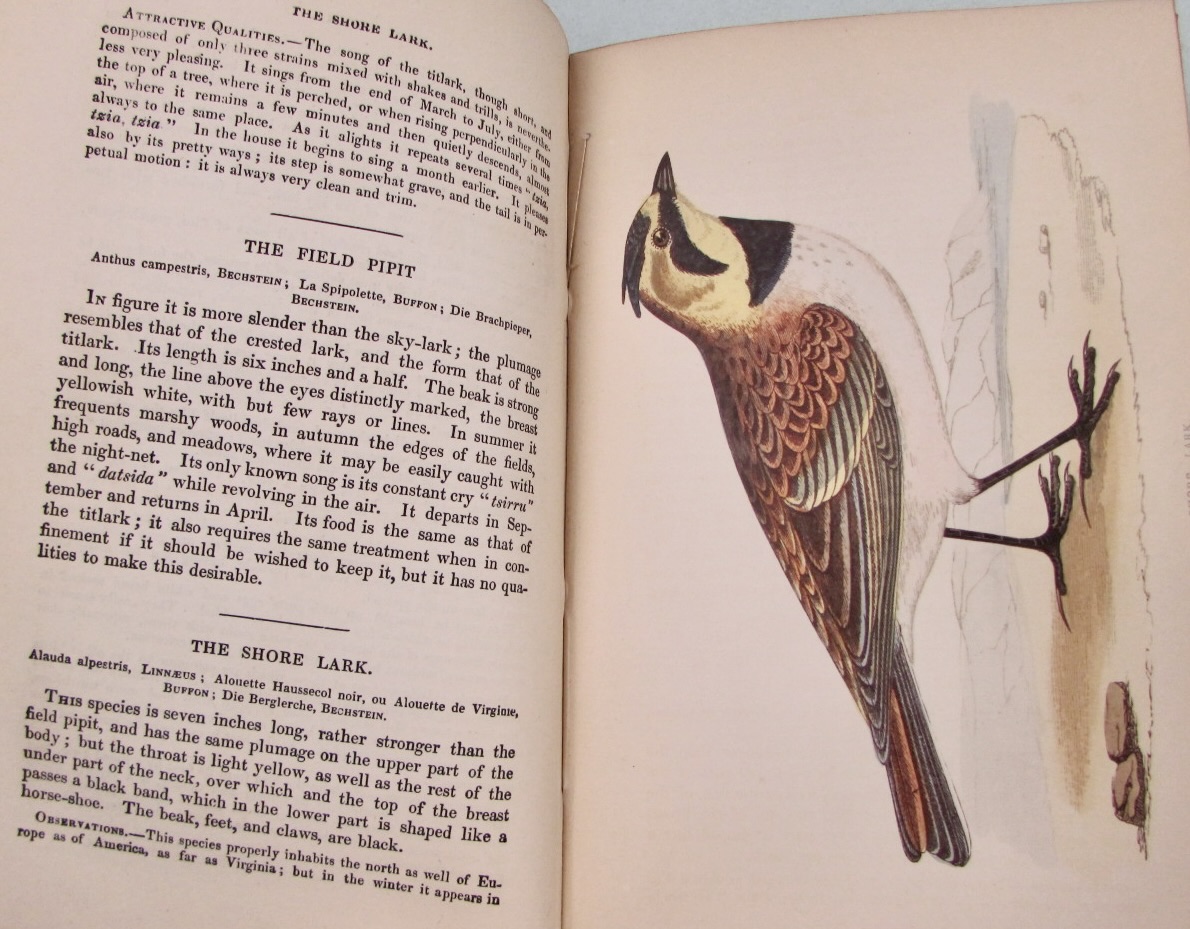The image depicts a page from an older book, possibly from the 1920s-40s, focused on birds. The open book features the left page filled with text divided into three distinct paragraphs, each separated by lines and titled "The Shore Lark," "The Field Pippet," and "The Shore Lark," suggesting detailed descriptions of these birds. The right page showcases a vertically oriented bird illustration. This bird stands on a white surface interspersed with rocks, against a backdrop that hints at water. The bird displays a complex coloration: its feathers exhibit various shades of brown, rust, light greenish, and beige; its belly is white; and its head is marked with black and yellow patterns. The bird also shows black striping on its neck and head. This intricate depiction highlights the bird's distinctive physical traits.